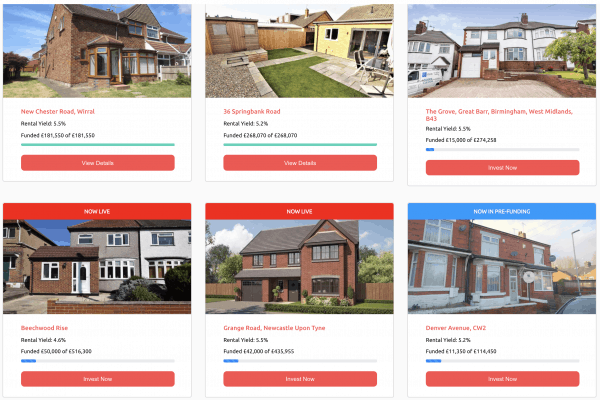This page features a detailed layout of six property listings arranged in two rows, each containing three properties displayed in square sections. Every square section includes a comprehensive set of property details along with a photo to provide visual context. 

In each square, the property photo is prominently displayed at the top, followed by the address of the property clearly stated. Information on the rental yield percentage and the current funding level for each property is also shown to help potential investors gauge investment viability. Below these details, a green progress indicator (likely representing the percentage of funding completed) is visible. Beneath the green line, there is a red rectangle containing white text which either prompts viewers to "View Details" or invites them to "Invest Now."

**Top Row:**
1. **First Property**: A brick, two-story building located on Newchester Road.
2. **Second Property**: A property under construction, primarily wooden, featuring a small yard and patio area.
3. **Third Property**: A two-story building situated at Grove Grape Bar, Birmingham, West Midlands.

**Bottom Row:**
1. **Fourth Property**: A two-story, brick building.
2. **Fifth Property**: Another two-story, brick building.
3. **Sixth Property**: Yet another two-story, brick building.

Each description is aimed at providing potential investors and viewers with a clear, informative, and enticing overview of the property opportunities presented.